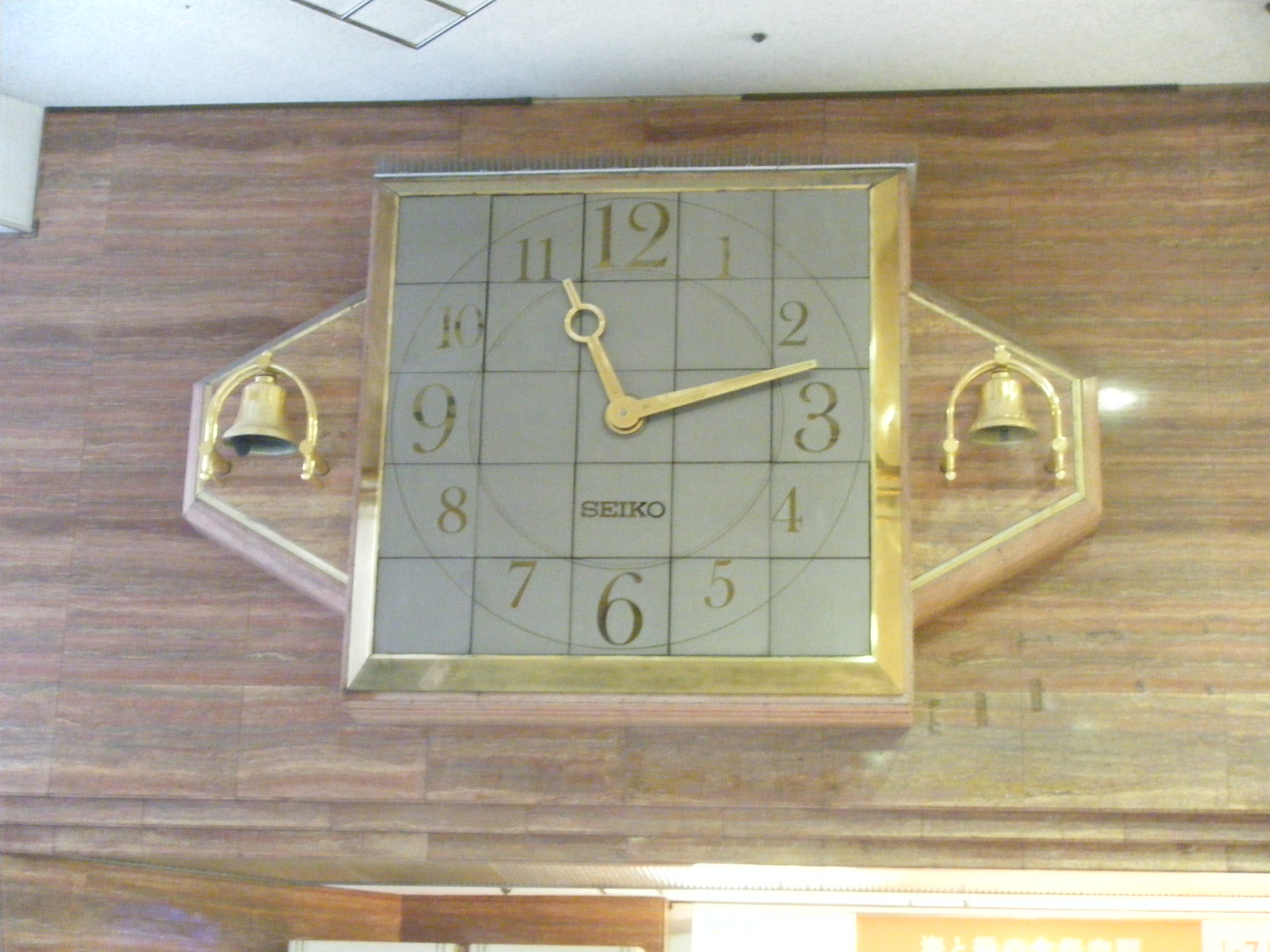This image, presented in a rectangular format with a horizontal orientation, has a vintage aesthetic characterized by muted colors and an overall aged appearance. Resting on a background that resembles a textured maple wood table is a square, gold-colored clock adorned with two small, gold bells positioned symmetrically on its right and left sides. The clock features gold hour and minute hands and a face marked by numeric hour indicators from 1 to 12, arranged clockwise. At the center of the clock face, just below the meeting point of the hands, is the brand name "Seiko," inscribed in small, gold capital letters. This timeless piece evokes a sense of nostalgia and classic elegance.